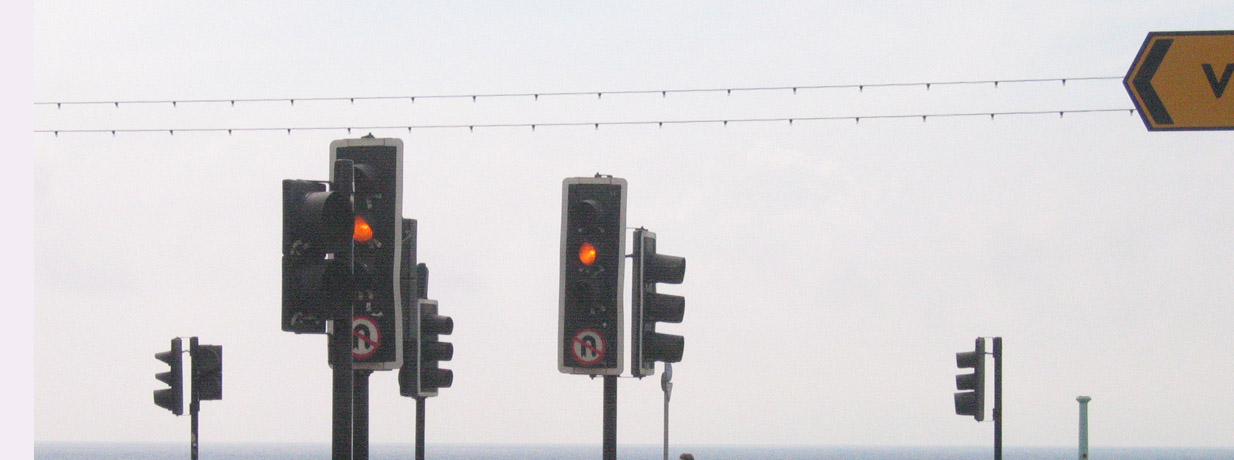This photograph, taken in a landscape orientation about three to three and a half times wider than it is tall, features a hazy, grayish-blue sky with a white overcast and clouds. Running horizontally about 20-25% down from the top, there are several power lines spanning the width of the image. On the upper right side, there is a yellow traffic sign adorned with a black left-pointing arrow and the letter "V", which appears to have a pointed edge with a black trim.

Dominating the lower half of the image are six pairs of traffic lights. The first, third, fifth, and sixth lights are oriented sideways, while the second and fourth traffic lights are facing head-on. All lit traffic lights currently show a red signal, and the two front-facing lights are uniquely marked with a white circle featuring a red line through it and a black letter “R”. Additionally, the lights themselves are outlined in white against a black background. The bottom right corner displays a green metal pole standing next to one of the traffic lights.